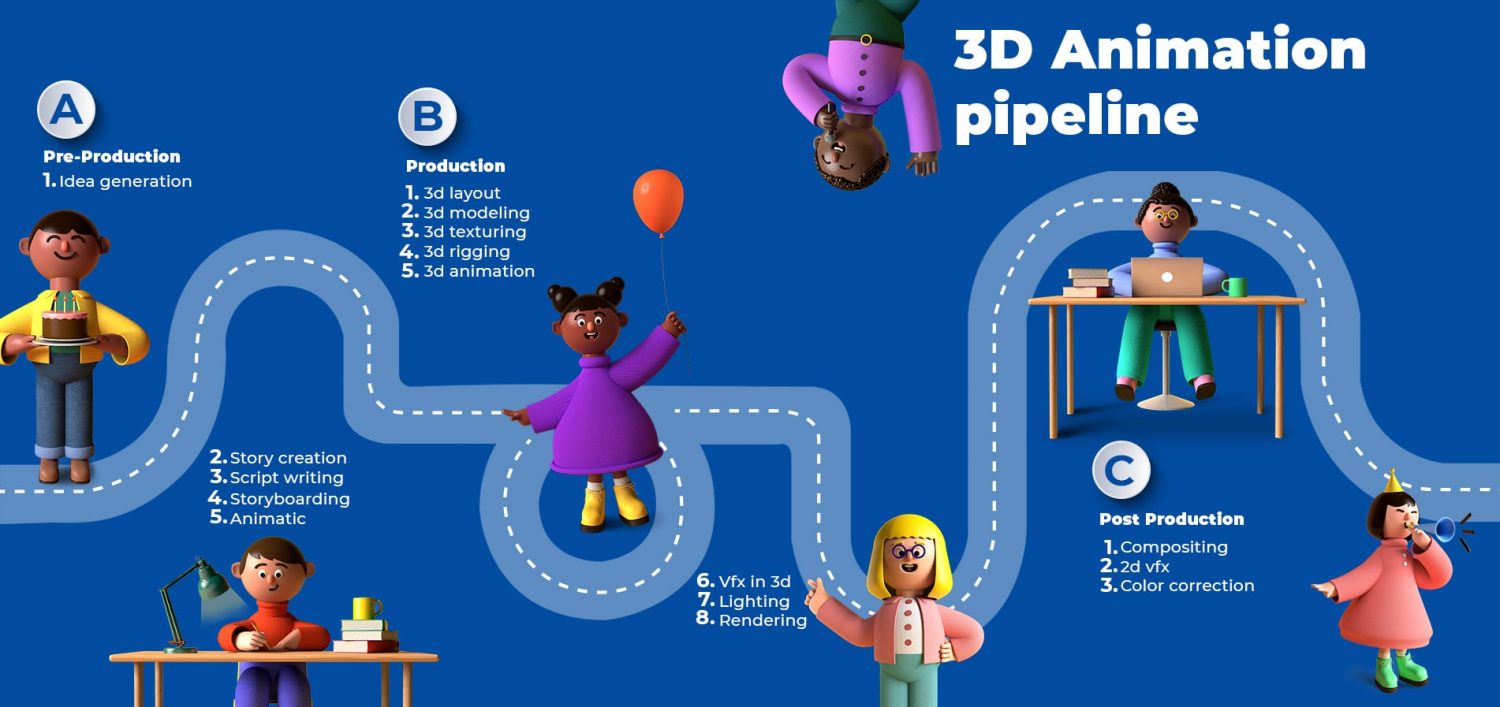The animated slide titled "3D Animation Pipeline" features a colorful, claymation-inspired visual representation of the animation process, divided into three main stages: Pre-Production (A), Production (B), and Post-Production (C). The title is prominently displayed at the top of a blue background rectangle. Below, a dotted road labeled A, B, C serves as the central path, guiding viewers through the stages, punctuated by a series of claymation figures that symbolize different parts of the process.

At point A, representing Pre-Production and idea generation, stands a smiling man in a yellow shirt and dungarees, holding a birthday cake. Next along the road is a person seated at a desk cluttered with a desk lamp, books, and a coffee cup, clad in an orange shirt and dungarees; this figure is engrossed in writing or sketching.

Point B showcases the Production stage, starting with an Afro-American girl with pigtails, wearing a purple dress and holding an orange balloon. Following her is a woman with blonde hair, bangs, glasses, and a pink cardigan, raising her hand with a somewhat intense expression. Nearby, an African-American woman works at a desk, using an Apple computer, surrounded by books and a green coffee mug.

At Point C, marking Post-Production, a girl in a peach dress with green Doc Martens and a triangle party hat is blowing a horn, resembling a birthday celebration. Above all these characters, in the upper section of the image near the title, an African-American boy in a purple shirt and green trousers hangs upside down, holding a microphone, possibly symbolizing the presenter of this animated journey.

The entire layout effectively tells the story of the animation pipeline through a creative and vibrant series of claymation characters, each adding to the narrative of moving from initial idea to final celebratory completion.